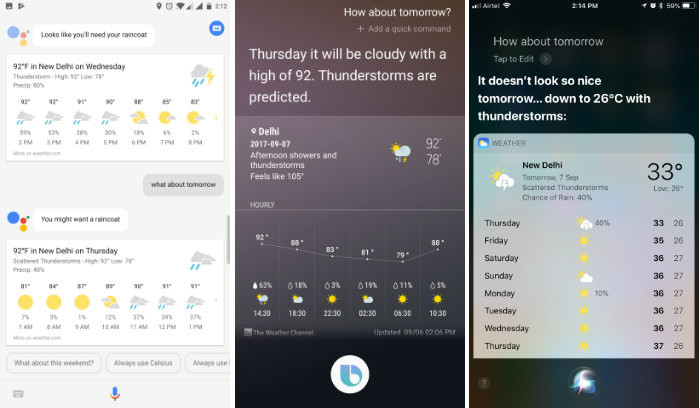The image features three different screenshots of weather forecasts displayed on various mobile phones, each representing different brands and interfaces.

**Left Phone: Google Pixel**
- The left screenshot appears to be from a Google Pixel device, displaying a detailed weather forecast for New Delhi. It advises, "Looks like you'll need your raincoat," with a temperature forecast of 92°F on Wednesday. It highlights thunderstorms with a high of 92°F and a low of 78°F, alongside an 80% chance of precipitation. The hourly weather breakdown from 2 PM to 8 PM shows icons indicating rain, overcast skies, and partly cloudy conditions. The top right of the screen features a larger storm icon and a query for the next day's weather, showing a similar forecast of rain and thunderstorms for Thursday.

**Middle Phone: Unknown Brand**
- The middle screenshot, from an unspecified phone brand, also provides a weather forecast for New Delhi. It indicates that "Thursday will be cloudy with a high of 92°F," predicting thunderstorms and afternoon showers. The feels-like temperature is a scorching 105°F, with the high and low mirroring the other forecasts at 92°F and 78°F respectively.

**Right Phone: Apple iPhone**
- The right screenshot depicts an Apple iPhone weather app with forecast information in Celsius. It predicts a drop to 26°C with thunderstorms for tomorrow in New Delhi. The current temperature is shown as 33°C. Notably, this forecast differs somewhat from the Google Pixel's, showing less stormy conditions and more sun for the coming days.

Overall, while each phone presents the information with its unique style, all three predict similar weather patterns involving warm temperatures and likely thunderstorms for New Delhi.